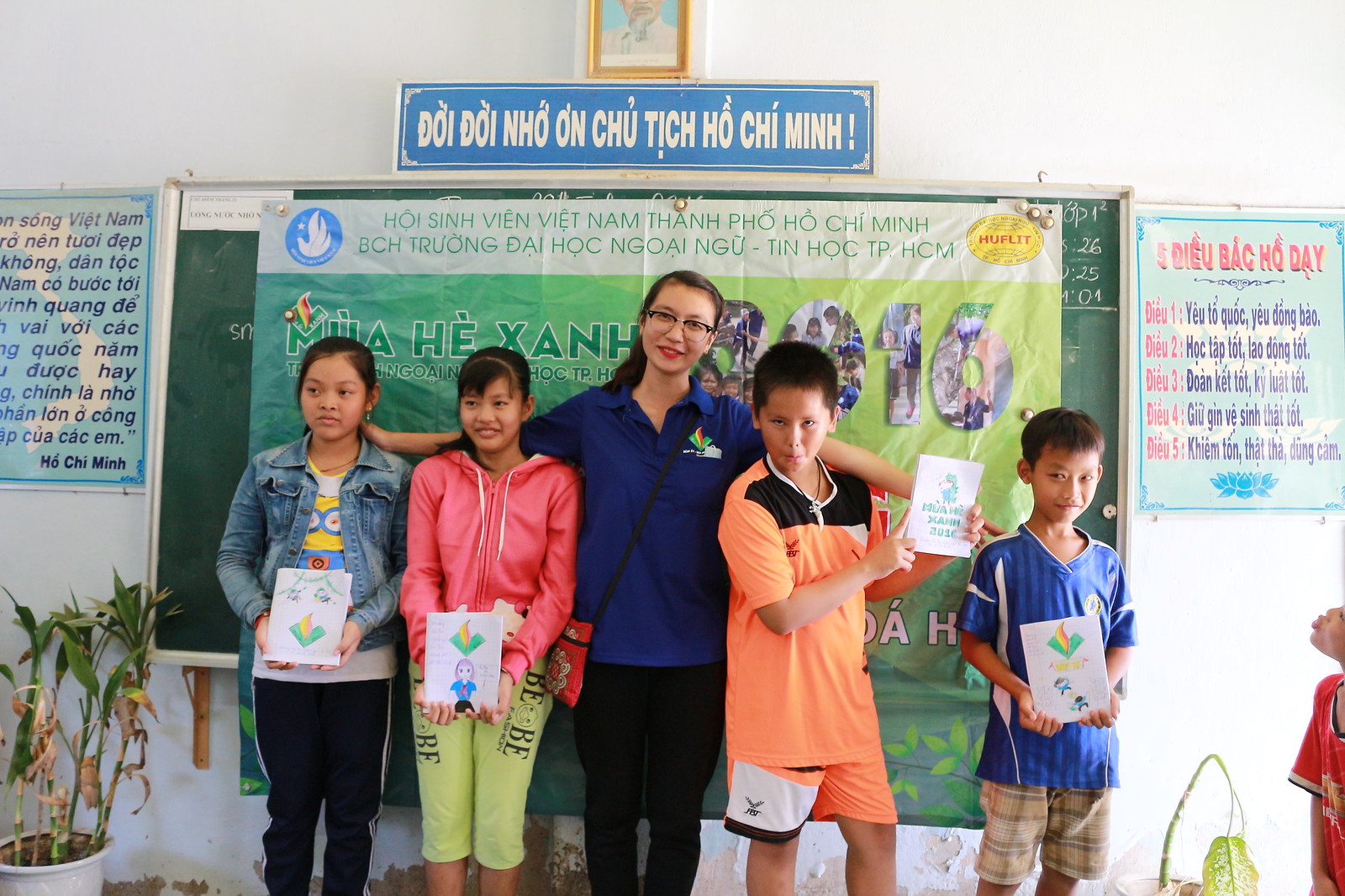The photograph captures a lively classroom scene during the daytime, illuminated by natural light coming from the right. The backdrop features a white wall adorned with various educational materials, including a green chalkboard partially obscured by a banner written in Vietnamese, accompanied by a rectangular blue sign with white Vietnamese text above it. Vibrant posters and some plants add more color and life to the scene.

Positioned centrally is a teacher in a blue shirt and glasses, smiling directly at the camera, exuding pride. Flanking her are five students, presumably of East Asian descent. On her left are two young girls, one in a jean jacket and the other in a pink sweater. To her right stand two boys, one in an orange shirt and the other in a blue shirt, while a third boy slightly cut off in the bottom right corner makes a playful kissy face, looking up at the others. Each student proudly holds up a piece of artwork they have created, adding a creative touch to the classroom's inviting atmosphere. The setting is richly detailed with colors including white, yellow, gold, light blue, dark blue, green, yellow, red, orange, pink, purple, and gray.